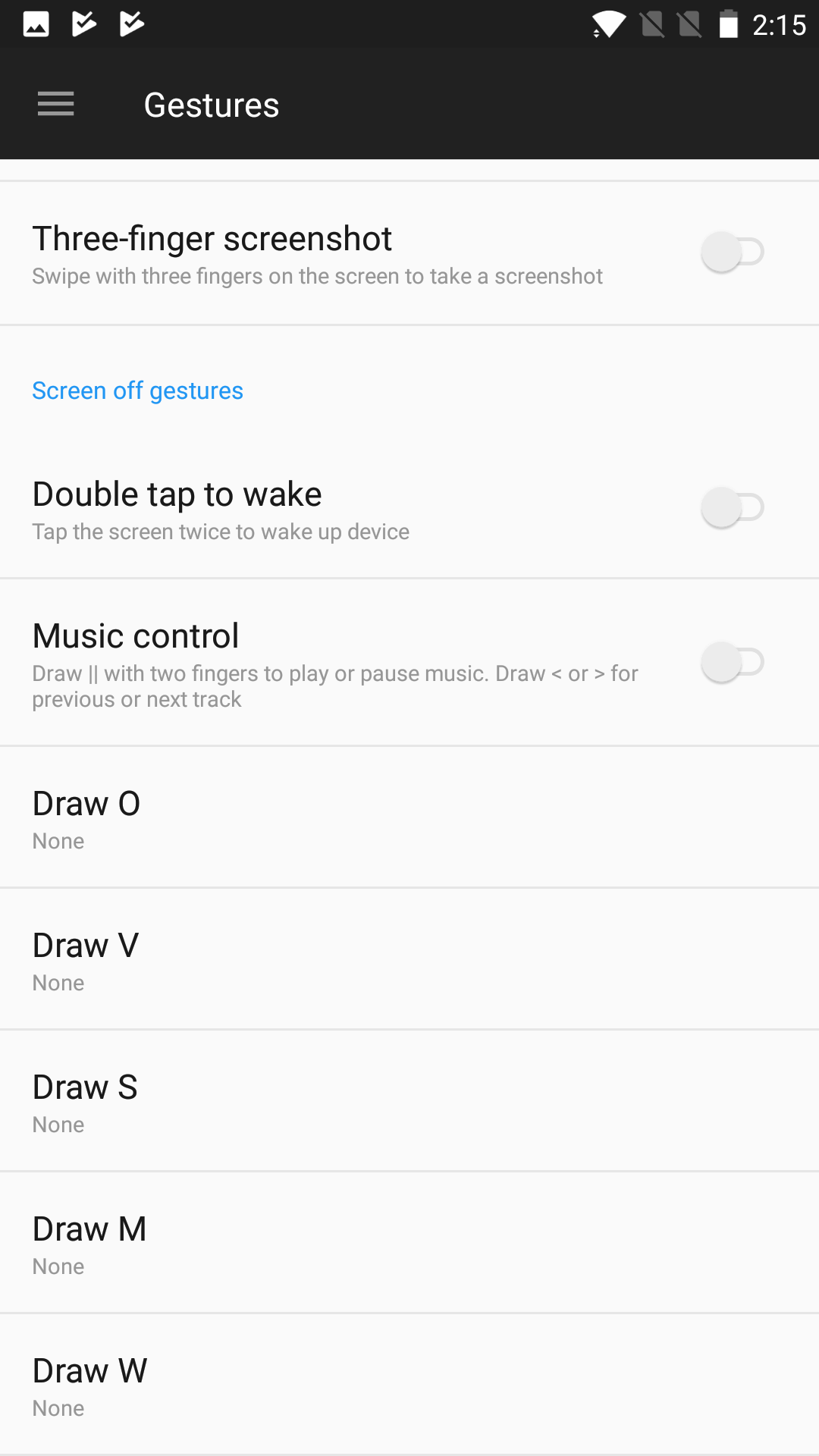This screenshot, taken on an Android device in dark mode, displays the Gestures section within the device's settings app. The interface lists several types of customizable gesture controls aimed at enhancing user interaction and accessibility. At the top, there's an option titled "Three-Finger Screenshot," accompanied by a description suggesting that swiping three fingers on the screen will capture a screenshot. Currently, this feature is disabled. Beneath this, the "Screen Off Gestures" option is listed, followed by the "Double Tap to Wake" feature, which can wake the device by tapping the screen twice, though this option is also not enabled. Further down, the "Music Control" feature advises users to draw two fingers on the screen to play or pause music. These gesture settings, likely part of the device's accessibility features, aim to improve usability for individuals with disabilities, including those with hearing, visual, or learning impairments.